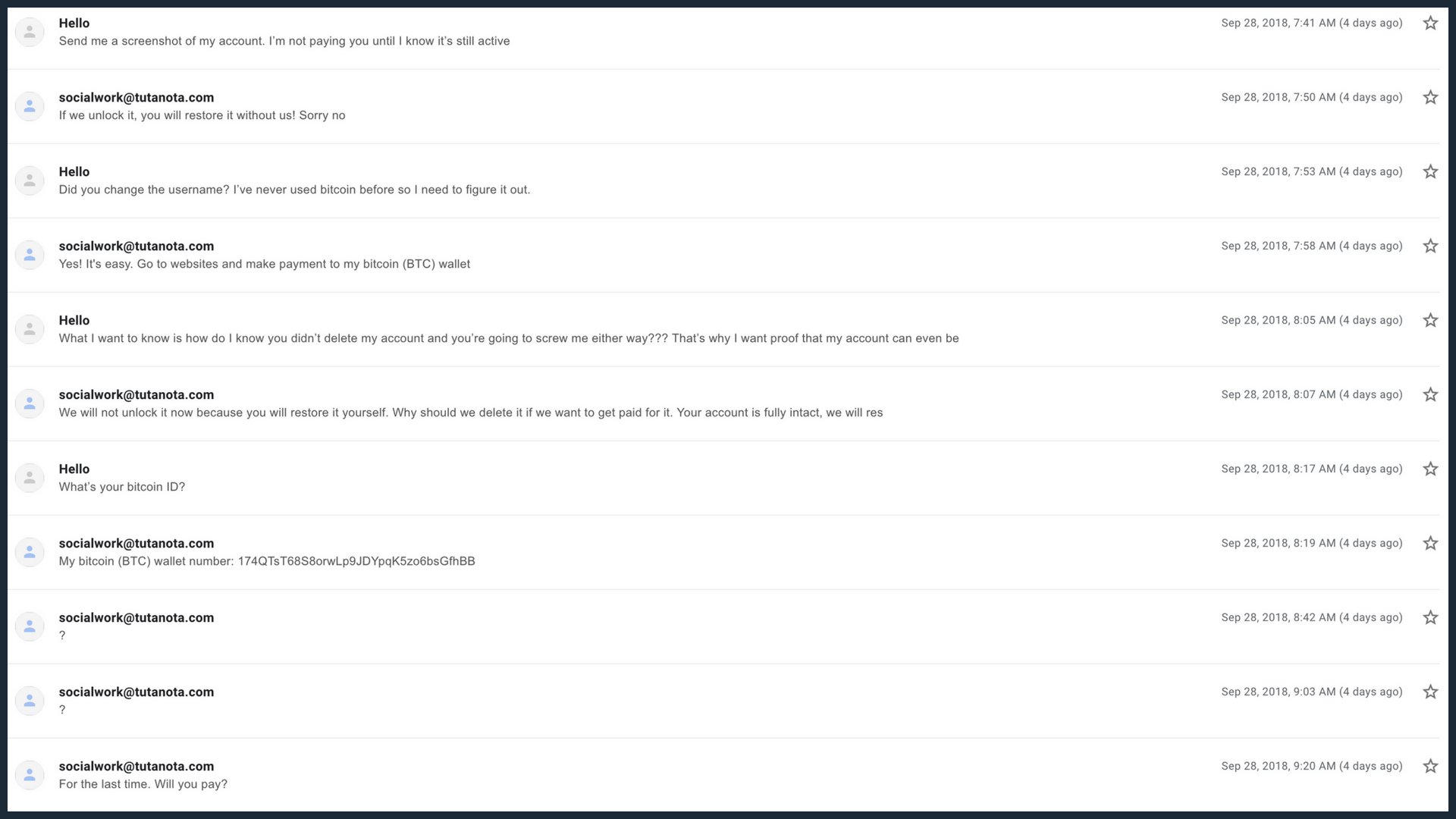**Detailed Caption:**

The image captures a chain of emails exchanged through Gmail, showcasing a correspondence regarding an account issue and payment conditions. The first email, dated September 28, 2018, at 7:41 a.m., has the subject line "Hello" and reads: "Send me a screenshot of my account. I'm not paying you until I know it's still active." This email is marked with a star icon on the right.

The subsequent response, from Social Work at Tutanota.com, dated the same day at 7:50 a.m., states: "If we unlock it, you will restore it without us. Sorry, no."

A follow-up email, dated September 28, 2018, at 7:53 a.m., inquires: "Hello, did you change the username? I've never used Bitcoin before, so I need to figure it out."

The next message, in a light gray font, dated 7:58 a.m. on the same day, responds: "Yes, it's easy. Go to websites and make payment to my Bitcoin (BTC) wallet."

At 8:05 a.m., a distressed email asks for assurance with multiple question marks: "Hello, what I want to know is how do I know you didn't delete my account and you're going to screw me either way??? That's why I want proof that my account can even be..." This message is truncated, cutting off mid-sentence.

The last visible reply, dated September 28, 2018, at 8:07 a.m., partially reads: "We will not unlock it now because you will restore it yourself. Why should we delete it if we want to get paid for it? Your account is fully intact. We will R-E-S..." and it also ends abruptly.

Each message is timestamped four days prior to the date of viewing, providing a clear timeline of the conversation.